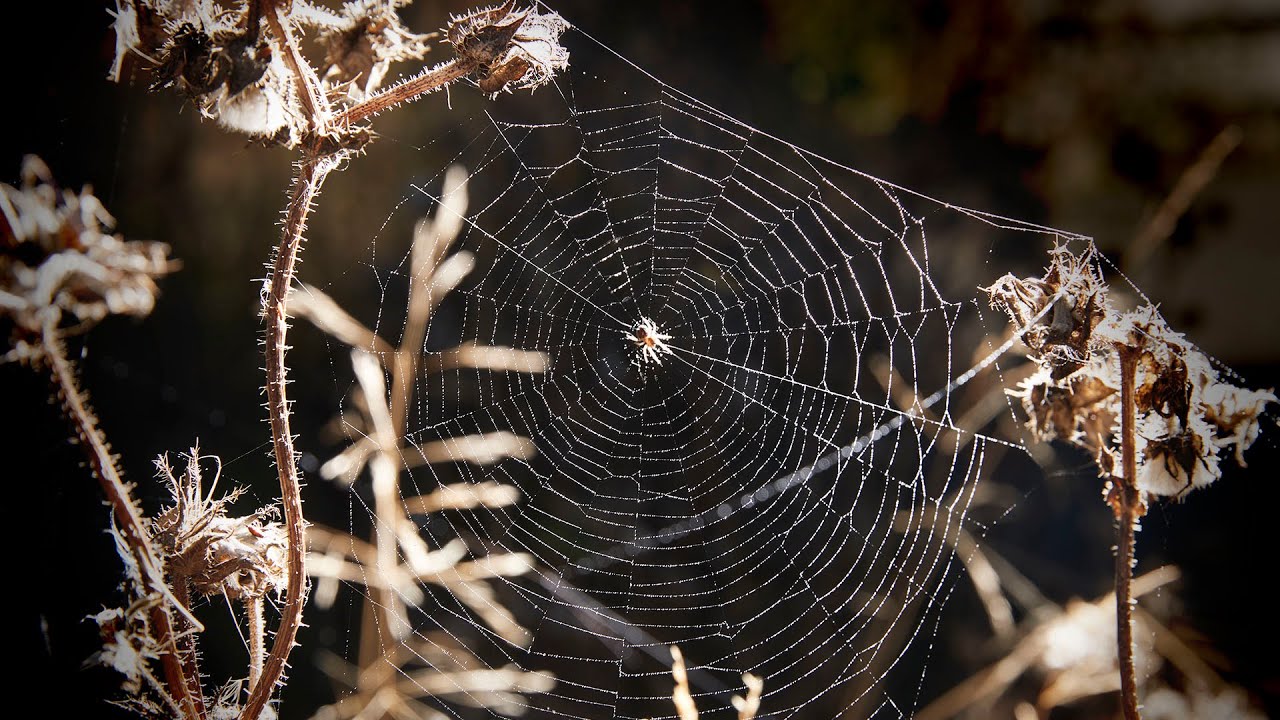This image showcases an intricately woven spiderweb positioned between two fuzzy-stemmed plants, resembling either cotton plants or dandelions, which could be dead or drooping. The spider is prominently centered within its finely detailed and circular web, appearing well-lit from behind by the light source, which enhances the vivid details of the spider and the web. The background fades into a soft bokeh, allowing the meticulous structure of the web to stand out. A single strand of the web extends forward, connecting to one of the plants, which is slightly out of focus and somewhat distracting. Despite this, the overall framing captures the spider perfectly, highlighting the delicate craftsmanship of its web against the subtle backdrop.